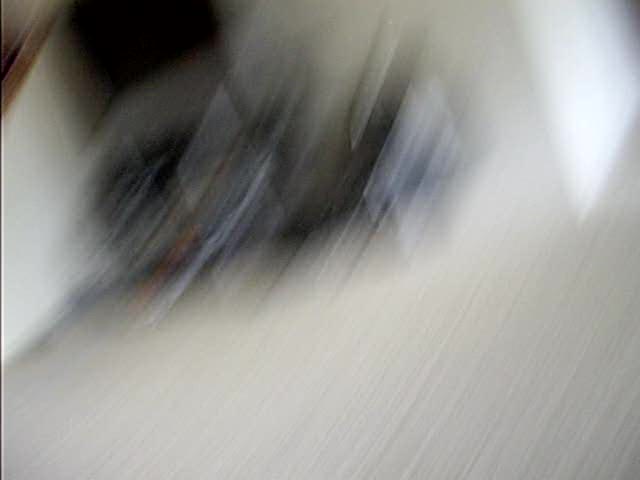This photograph appears to be taken inside a living room, characterized by white flooring and a black entertainment center positioned against the far wall. On the left side of the image, there is a wall that might be part of a stairway descending or ascending. However, the entire scene is enveloped in motion blur, as if the camera was in swift movement when the picture was taken. The resulting blur lines cascade from the top of the image to the bottom, curving upwards to the left, creating an abstract, almost dynamic pattern that obscures the details of the room.